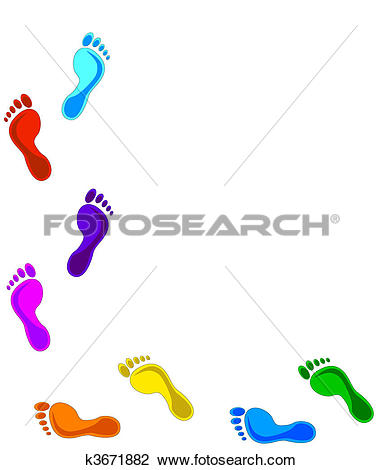The image appears to be a digitally created advertisement or logo for a company named PhotoSearch. It features a series of eight colorful clipart-style footprints, arranged in pairs and moving diagonally from the bottom right to the top left. The footprints, depicted in vibrant shades such as green, blue, yellow, orange, magenta, dark violet, red, and a bright turquoise, traverse across a faint gray X watermark that spans the entire background. At the intersection of the X, the company's name "PHOTOSEARCH" is prominently displayed in gray, capital letters. Beneath this, the identifier "K3671882" and the website URL "www.photosearch.com" are printed, providing additional company information. The design suggests a modern, playful aesthetic, potentially aimed at a photo clipping or stock image service.